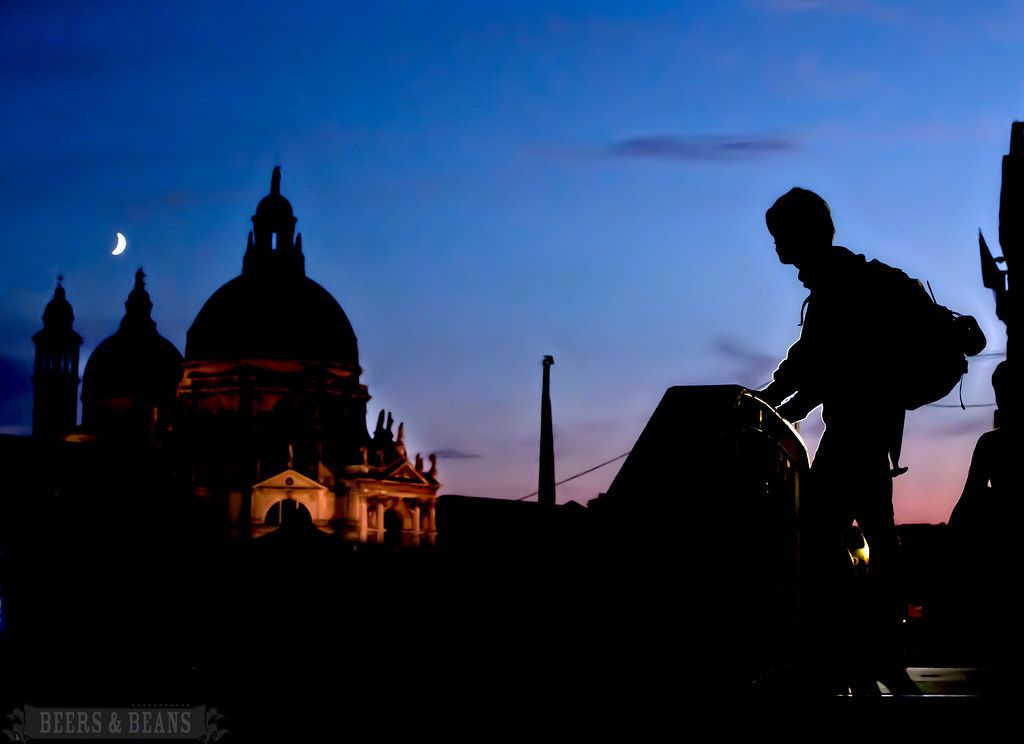The image depicts a serene evening or early dawn scene, likely set in India, with a striking display of architectural beauty reminiscent of domed buildings like the Taj Mahal. The backdrop is an enchanting blend of deep blue and purplish-red hues of the sky, gradually transitioning to a somber night with a faint crescent moon hanging in the upper left corner. The silhouette of a person, donned in a hooded jacket and carrying a backpack, walks towards the left side of the frame, shrouded in shadows that render finer details imperceptible. In the background, a notable building—possibly one among several—stands partially illuminated, contrasting against the silhouettes of its majestic structures, while the sign "beers and beans" is subtly visible in the bottom left corner. The scene exudes a tranquil and almost mystical ambiance, capturing a fleeting moment as daylight retreats or begins anew.